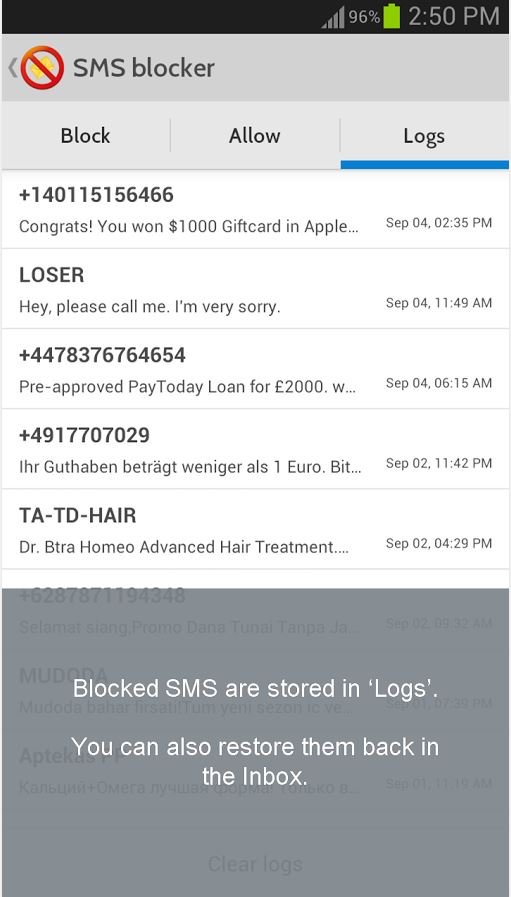This detailed caption describes the contents of a smartphone screenshot displaying an SMS blocker application:

---

The screenshot from a smartphone features the main interface of an SMS blocker app. At the top, a prominent red circle with a slash through it, along with an orange background, symbolizes the blocking function. Underneath this icon, three tabs labeled "Block," "Allow," and "Logs" are displayed horizontally in a gray bar, each tab separated by faint vertical lines.

Below these tabs, the intercepted messages are listed chronologically. The first message at the top displays a sender's phone number starting with a plus sign, followed by the message preview: "Congrats, you won $1,000 gift card in Apple..." accompanied by the date and time, "September 4th, 2:35 p.m." 

The subsequent message, also dated September 4th but at 11:49 a.m., is more abrupt, shouting in capital black letters: "LOSER. Hey, please call me, I'm very sorry."

Three additional blocked messages follow, each with corresponding dates and times.

At the bottom of the screen, a noticeable gray box with white text informs the user: "Blocked SMS are stored in logs. You can also restore them back in the inbox."

---

This caption provides a thorough and descriptive overview of the visual elements and textual content present in the screenshot.